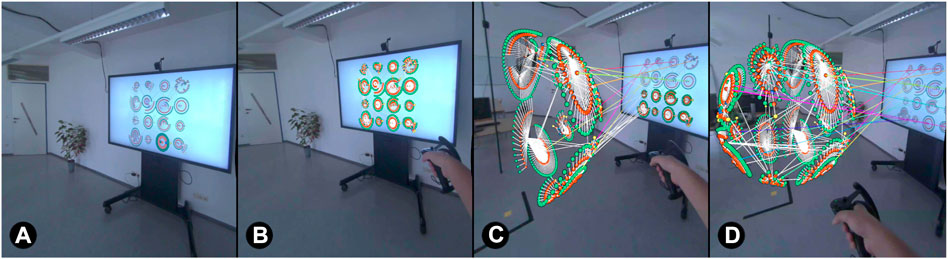The series consists of four images labeled A, B, C, and D, all set in a consistently depicted room with plain white walls, a darker gray floor, a potted plant, a door to the left, and a freestanding TV or computer screen on wheels to the right. In the first image (A), the screen displays 16 geometric elements on a white background. The second image (B) shows a glowing screen with these elements becoming more vibrant and a hand entering the frame from the right, holding a controller. In the third image (C), the top six colorful elements – green, orange, and white – leap off the screen, appearing in midair with strings connecting them back to the screen, creating a 3D effect. Finally, in the fourth image (D), these elements have morphed into a spherical arrangement of spiky, colorful shapes, now forming a floating, dynamic 3D structure, with the hand still holding the controller, suggesting manipulation of the digital projections into virtual reality.